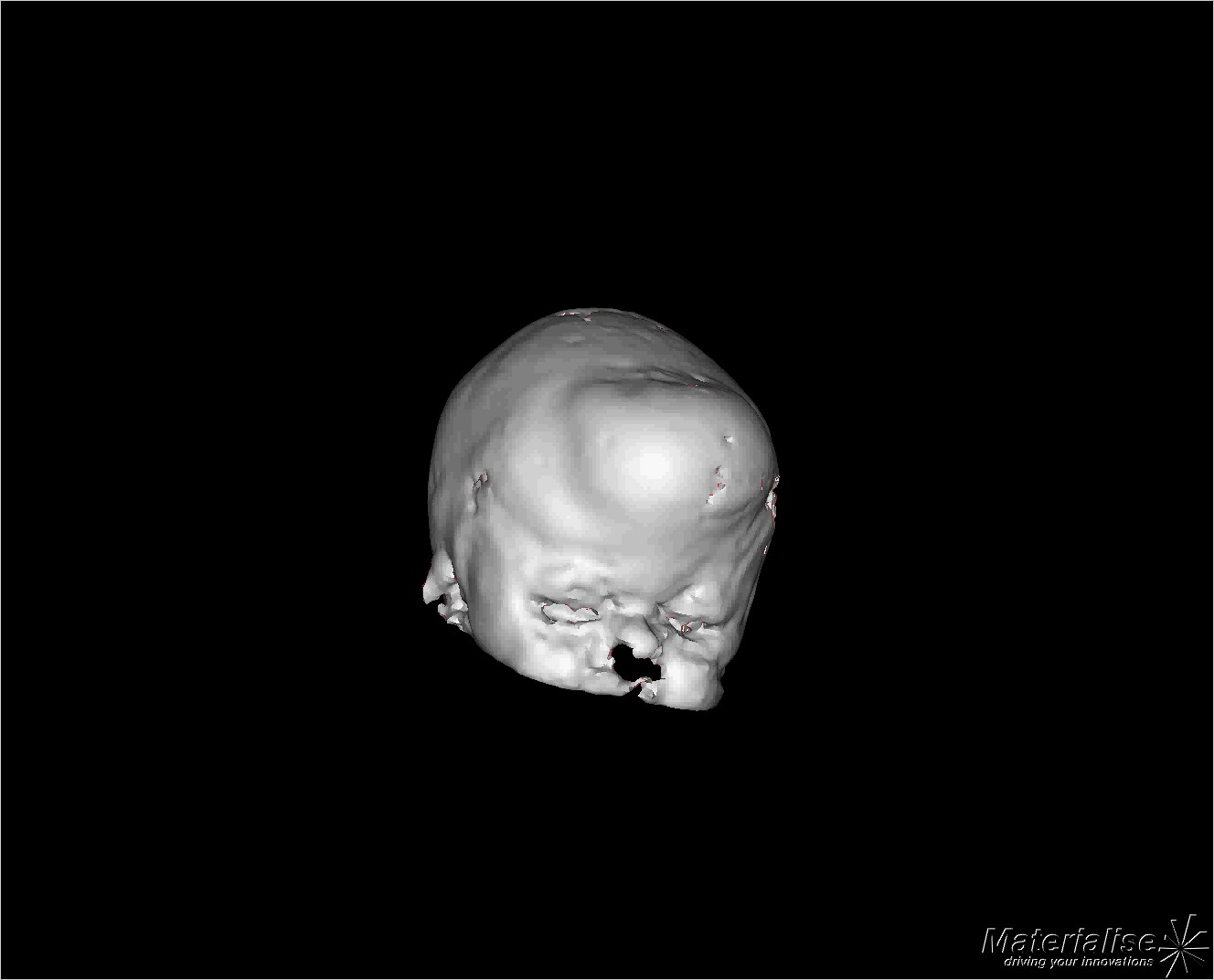The image appears to be a high-resolution 3D scan of an infant's skull, likely created using advanced imaging technology from a company named Materialize, as indicated by their logo and tagline "Driving Your Innovation" in the bottom right corner. The skull is depicted with notable clarity, showing both bone and flesh, though the image is limited to the area above the nose. The forehead has a prominent, dome-like protrusion, which may suggest a deformity; this, however, could also be an artifact of the 3D rendering process. The scan features unusual holes in the skull, including a notable one around the nasal area, and the entire depiction is set against a pitch-black background.